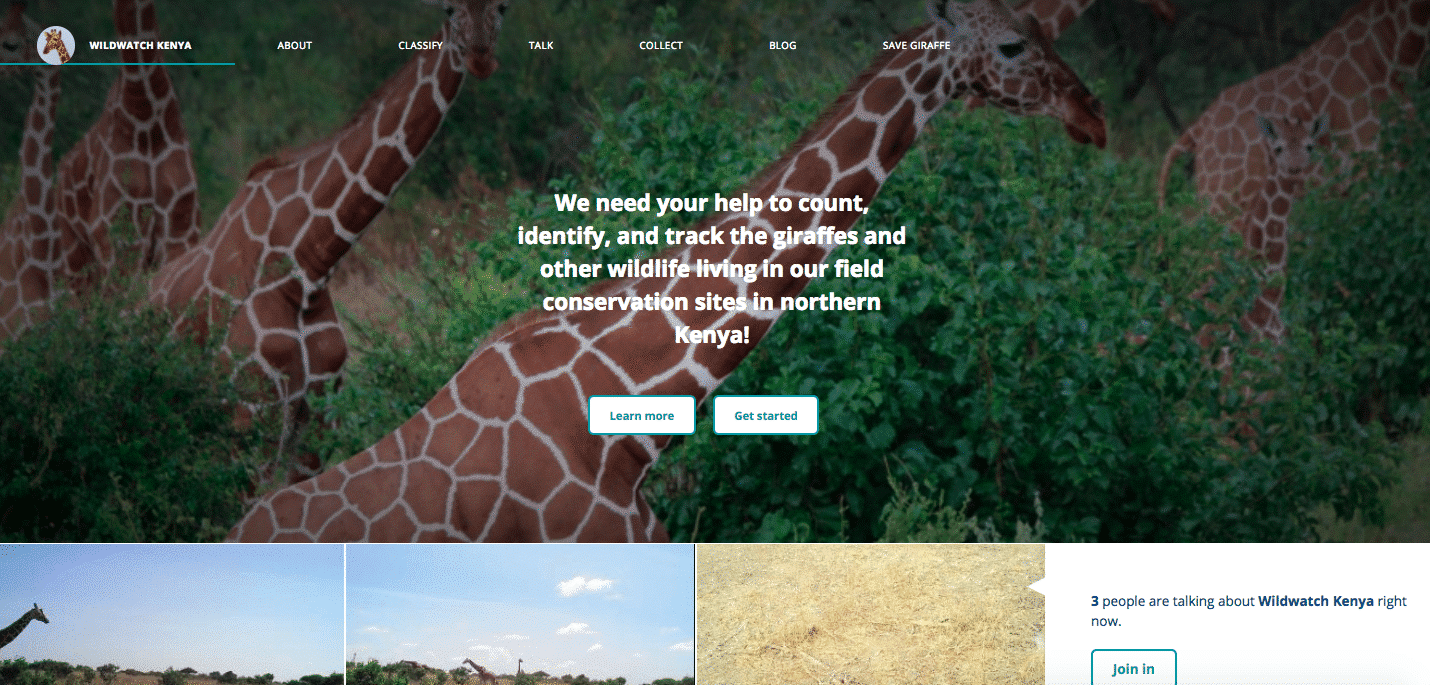The screenshot from the Wild Watch Kenya website prominently features a vibrant call-to-action layout. In the top left corner, the site’s logo is displayed alongside a charming circular image of a giraffe. A horizontal menu offers various site navigation options: About, Classify, Talk, Collect, Blog, and Save Giraffe.

Dominating the page is a full-width image showcasing a group of four giraffes. These giraffes, notably darker brown than the usual yellow, grace the landscape of northern Kenya. A call-out message appeals for help in counting, identifying, and tracking these giraffes and other wildlife within the conservation sites. 

Beneath this call-to-action, two buttons invite further engagement: "Learn More" and "Get Started", set in white boxes with green borders. At the page's bottom, a trio of smaller images is displayed: one showing a solitary giraffe against the sky, another depicting a distant herd, and a third, unclear image, possibly of the terrain. A footer note reads, "Three people are talking about Wild Watch Kenya now. Join in."